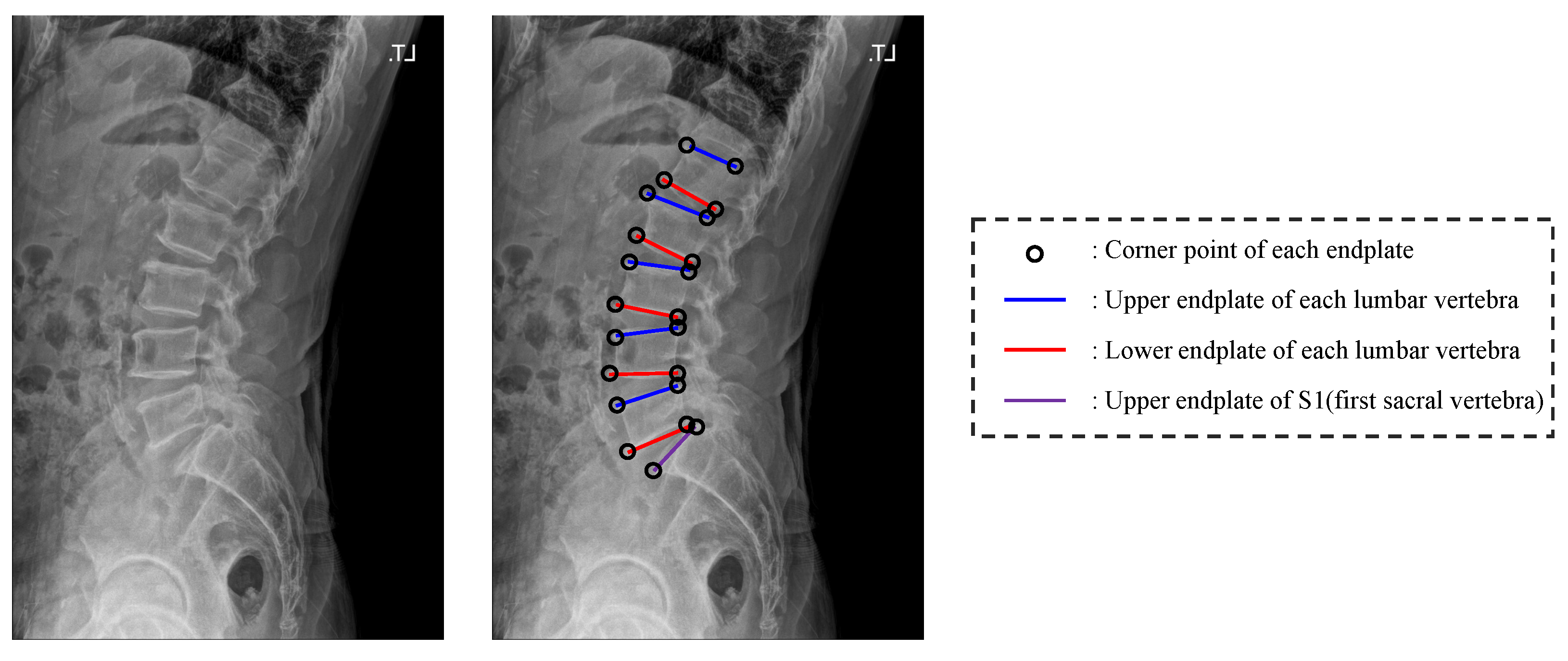The image set consists of two X-rays displayed side-by-side in a vertical, portrait orientation, focusing on the side view of a person’s torso from the chest to just below the glutes, emphasizing the spinal column. Both images have the identifier "TJ" in white font at the top right corner. The left image is a plain X-ray, while the right image is annotated with multiple colored lines and black dots: the blue lines denote the upper end plates of each lumbar vertebra, the red lines indicate the lower end plates of each lumbar vertebra, and the purple line represents the upper end plate of the first sacral vertebra (S1). Each line's endpoint is marked by black circles denoting the corner points of each end plate. A dotted black rectangular box on the far right provides a legend explaining these color codes and symbols. At the top, the pattern alternates between blue and red lines down the spine, with the very bottom exhibiting the lone purple line.